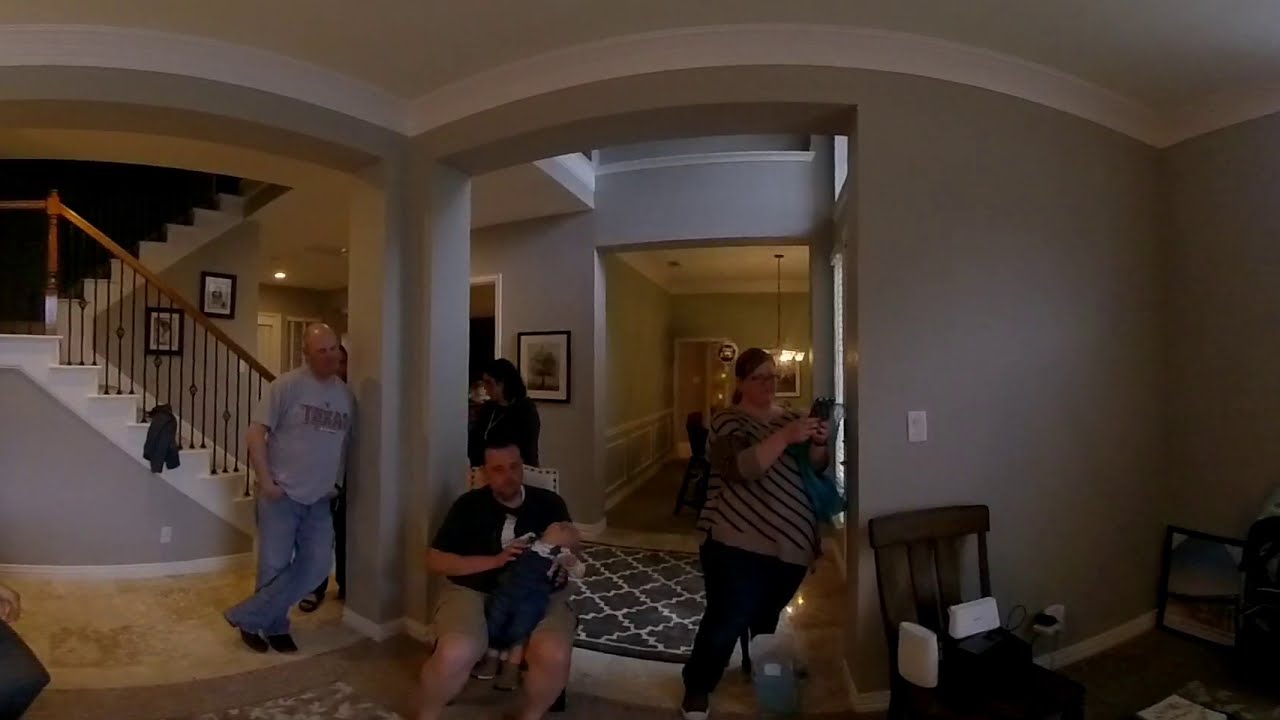The image captures an indoor scene of a residential home with a split staircase on the left, angling up to the left before turning back to the right. The staircase area is highlighted by a light marble floor at its base. Adjacent to the staircase stands a pillar, against which a bald middle-aged Caucasian man in a gray t-shirt and blue jeans is leaning. On the right side of the pillar, a younger overweight Caucasian male with short dark hair sits in a chair, wearing a black shirt with a white emblem and light-colored shorts, holding a blue item in his lap. Standing further to the right is a middle-aged, overweight Caucasian woman with dark hair in a ponytail, glasses, and a striped tan shirt paired with dark pants. She holds a phone and looks forward, slightly to the right. Behind her and the seated man, a woman with shoulder-length dark hair, dressed in dark clothing, can be seen near a hallway. This hallway leads to a foyer filled with natural light, transitioning to a formal dining room with green walls and a glass china cabinet. The living space in the foreground has gray walls with white borders and features scattered area rugs, a framed object in the corner, and a mix of carpet and marble flooring, suggesting a well-furnished, albeit dimly lit, daytime setting.